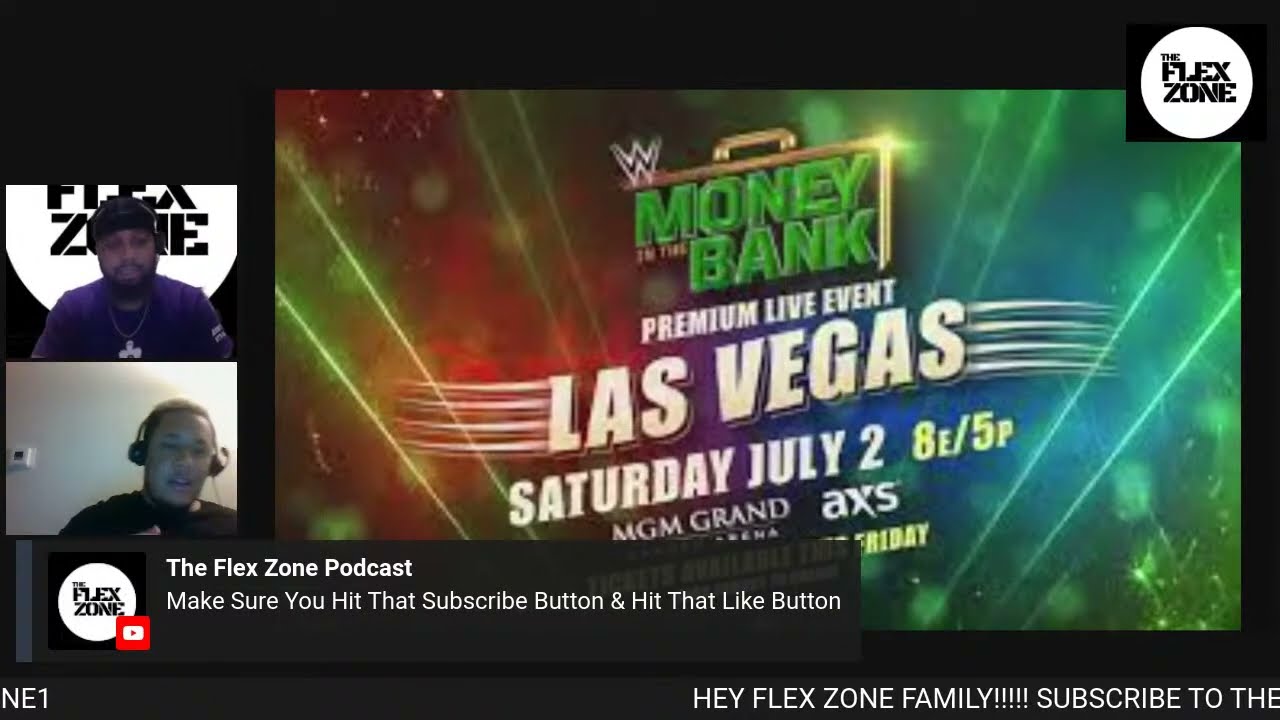The image features an intricate advertisement for the WWE "Money in the Bank" Premium Live Event scheduled for Saturday, July 2nd, in Las Vegas at the MGM Grand, with the broadcast times of 8E/5P, prominently displayed in green and yellow fonts. The banner, set against a black background, emphasizes the event details in white font, with an additional note of "AXS" beneath it. 

The top right-hand corner displays a white circle with the black text "The Flex Zone." Extending this branding, the bottom left corner reiterates the "Flex Zone" logo with a YouTube icon, and text urging viewers to "make sure you hit that subscribe button and hit that like button" in white font. Below, it reads "NE1," while the bottom right contains the greeting "Hey Flex Zone family!!! Subscribe to the."

On the left-hand side of the image, two YouTubers are featured in a vertical arrangement. The upper individual, a black man wearing a backwards black hat, blue shirt, silver chain with a pendant, and sporting a black beard, has a partially visible "Flex Zone" logo behind him. Below him, another black man in a black shirt and headphones is seen against a plain white wall with a thermostat, engaging with the content. The image captures their likely commentary and reactions to the wrestling event, adding an interactive dimension to the advertisement.